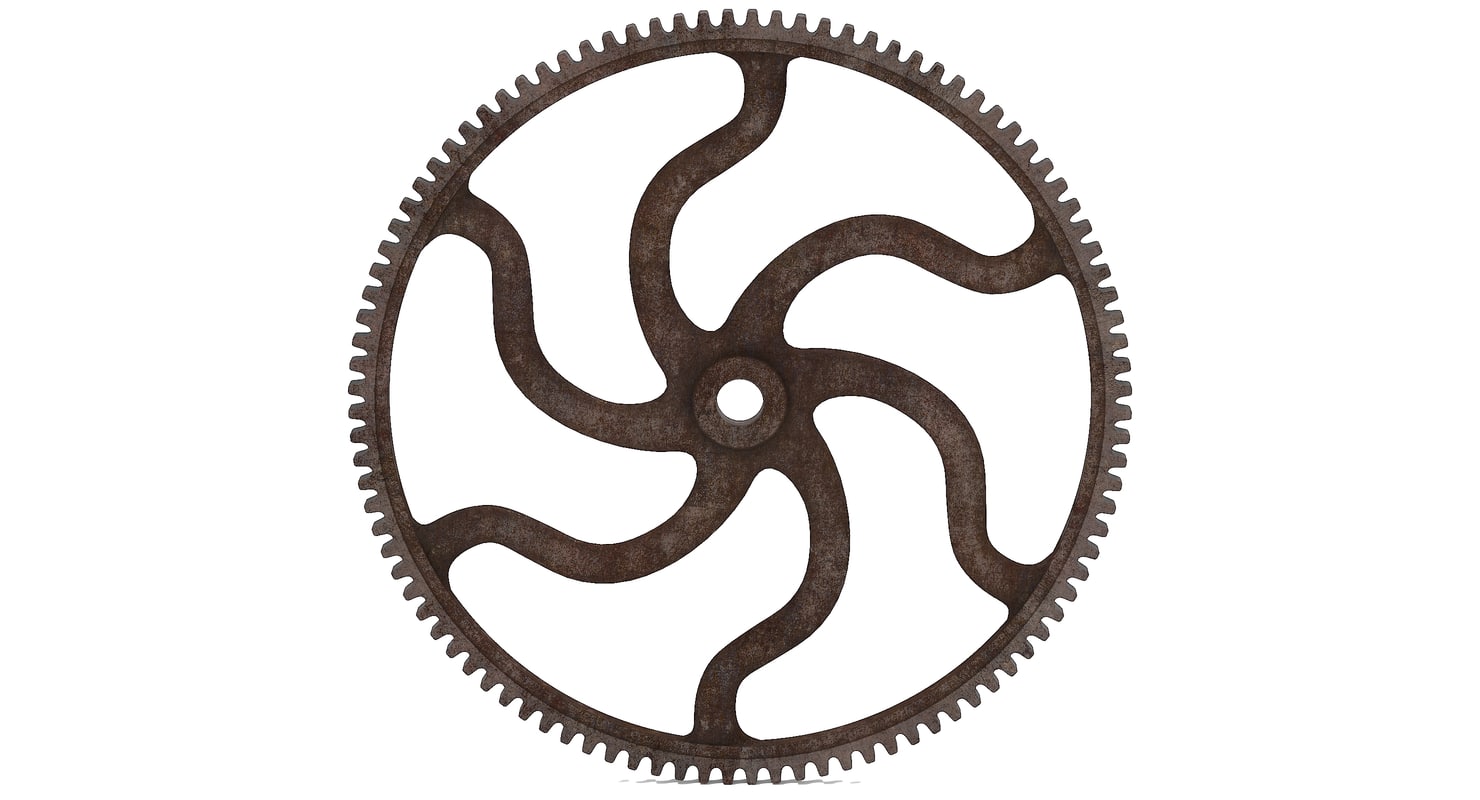The image showcases a large, detailed metal wheel centered against a completely white background. The wheel, which dominates almost the entirety of the image, appears to be made of dark metallic brown material. The structure consists of a round outer gear with evenly spaced teeth along its circumference. The focal point is the intricate center, featuring six wavy, squiggly connectors that radiate outward from a central hole. These connectors, reminiscent of an octopus's tentacles or a spider’s legs, create a spiraling effect within the wheel. The spaces between these wavy lines are white, enhancing their visual prominence. There is no text anywhere on the image, suggesting its use could be for a maintenance website, clipart, or an online image hosting service. The simplicity of the white and metallic color scheme and the precise details emphasize both the artistic and functional aspects of the wheel.